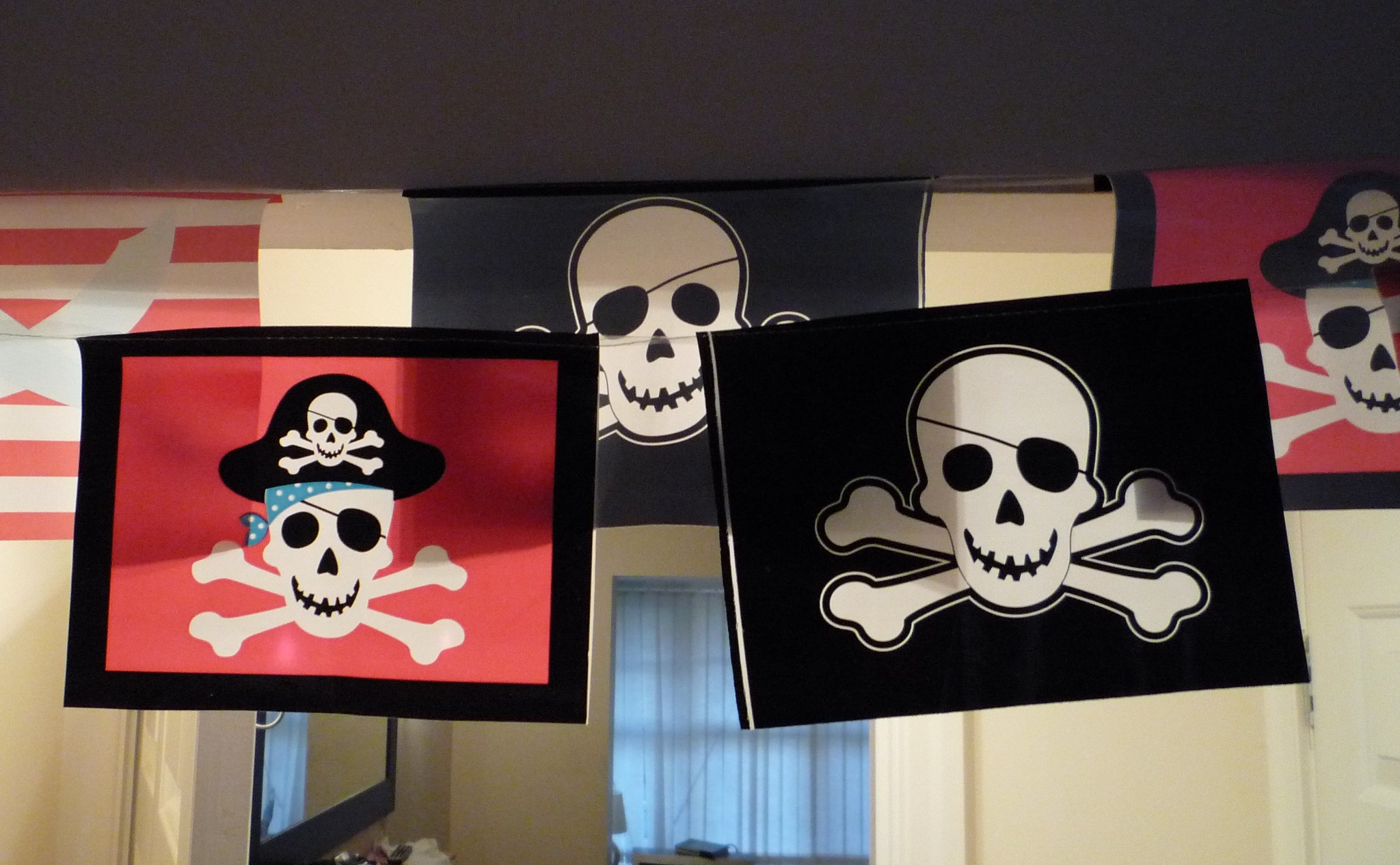The photograph features five intricately designed pirate flags hung from a gray cross beam near the ceiling of a room. The beam itself transitions from a dark gray on the top to a lighter gray on the underside. The flags range in size, with each featuring variations of skull and crossbones with pirate accents like eye patches, hats, and bandanas.

Starting from the top left, the first flag is adorned with red and white stripes and showcases two crossed swords. To its right, a black flag displays a white skull wearing a patch over its left eye and crossbones beneath. Further right, half-visible, is a red flag with a black border, depicting a skull with a similar eye patch, crossbones, and a black hat with another skull emblem.

On the second row, the flag to the left features a black border and a red interior, showcasing a skull with a blue bandana, an eye patch over its right eye, and a black hat adorned with skull and crossbones. The final flag is predominantly black with a white skull and crossbones, and it also carries an eye patch over the right eye.

The photograph captures the flags hanging against a backdrop of a white wall, with a doorway in the center framed by white trim. Through the doorway, a window with a curtain partially drawn allows in some light. On the left side, the bottom of a mirror with black trim is visible, while on the right, part of another door with white trim can be seen. The room is depicted from a high vantage point, emphasizing the ceiling and upper features.